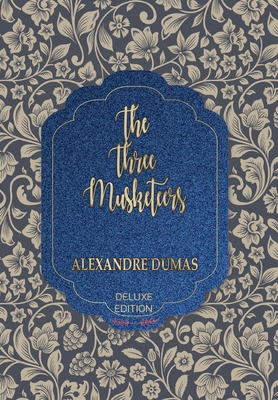The image depicts a highly detailed cover of the book "The Three Musketeers" by Alexandre Dumas. The cover features a dark gray, almost black, background adorned with an intricate pattern of white flowers and leaves. At the center of the cover, there is an ornately-shaped blue oval with a gold border. Within this blue oval, the book's title, "The Three Musketeers," is prominently displayed in large, fancy gold letters. Beneath the title, the author's name, "Alexandre Dumas," is written in smaller, regular gold letters. Additionally, the notation "Deluxe Edition" can be seen in white letters below the author's name. The overall image is clear, colorful, and appears to be well-lit with natural light, highlighting the intricate floral design and the decorative elements that frame the central title.